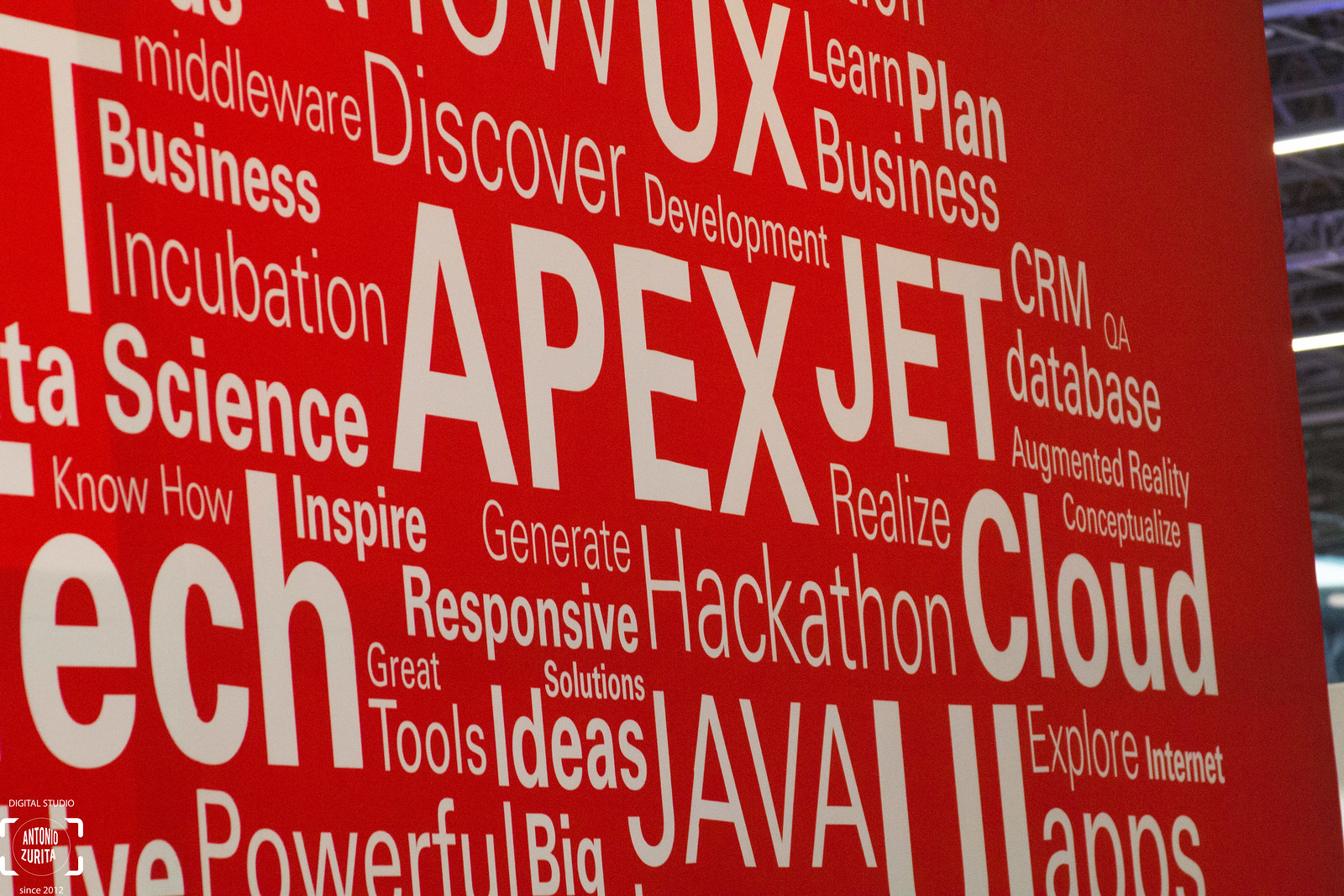The photograph features a vibrant red background densely populated with a word cloud composed of white text in varying fonts, sizes, and thicknesses. Some words are in all caps, while others are in lowercase, creating a dynamic visual effect. Due to the cropping of the image, some text appears partially cut off. Prominent words in the word cloud include "UX," "learn," "plan," "business," "discover," "development," "CRM," "QA," "database," "jet," "realize," "hackathon," "cloud," "responsive," "generate," "solutions," "tools," "ideas," "Java," "explore," "internet," "powerful," "big," "tech," "how-to," "science," "incubation," "middleware," "apex," "augment," and "reality." The arrangement suggests it might be promoting various tech concepts, tools, and methodologies, possibly as part of a tech advertisement or presentation board. In the background, elements of a meeting room, such as a section of the ceiling and some lights, are visible on the right, providing context that this display might be part of a conference or business event setup.